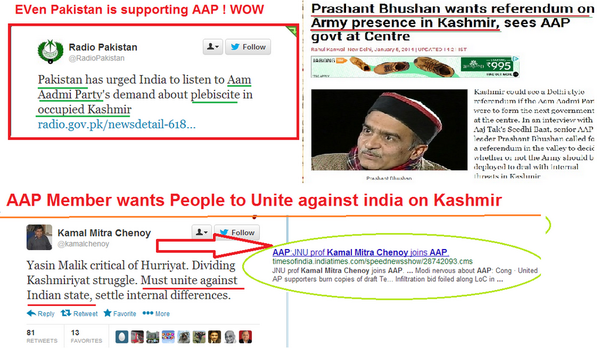The image is a collage of screenshots featuring several comments and an article. On the left side of the image, there are multiple comment screenshots. The first comment, located in the upper left corner, is highlighted with a red rectangular border. Above this comment, red text reads, "Even Pakistan is supporting AAP! Wow!" Directly below, another comment is seen, also marked with red text, stating, "AAP member wants people to unite against India over on Kashmir."

On the right side, a screenshot of an article is visible. The article's title is underlined in red and is written in black text. Below the title, a rectangular image of a man is displayed. The man is set against a black background, wearing a black and red hat and a black and red plaid scarf around his neck. He is also dressed in a light brown shirt.

A prominent red arrow points toward the right, directing attention to a blue link. Beneath this blue link, there is a green website link. The article includes a short description, written in black text, all of which is enclosed in a lime green oval border.